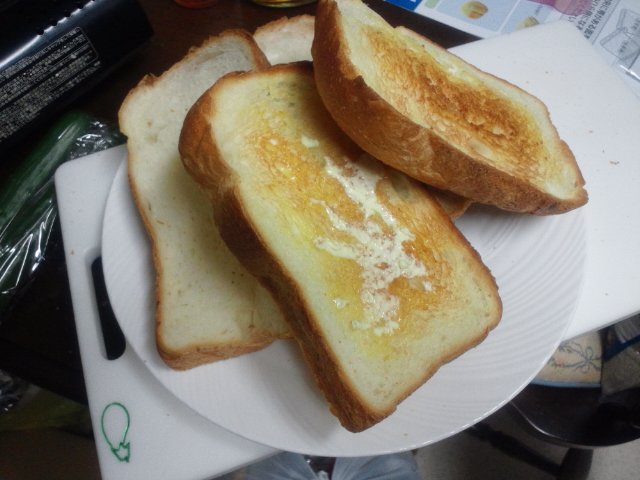This landscape-oriented color photograph presents a first-person perspective looking down at a white bone china plate holding several slices of toast. The plate, round in shape, features detailed ridges that sweep out from the center, mimicking a seashell design. Four pieces of toast are haphazardly piled, with the slice closest to us generously buttered. The topmost slice appears to be the heel, distinguished by its thicker top edge, while some in the background might be untoasted. 

Below the plate, a thick, white cutting board runs diagonally from the bottom left to the upper right, revealing an oval handle just to the left of the plate. Additionally, a green logo resembling a courgette is printed on the top left corner of the cutting board, adding a splash of color to the scene.